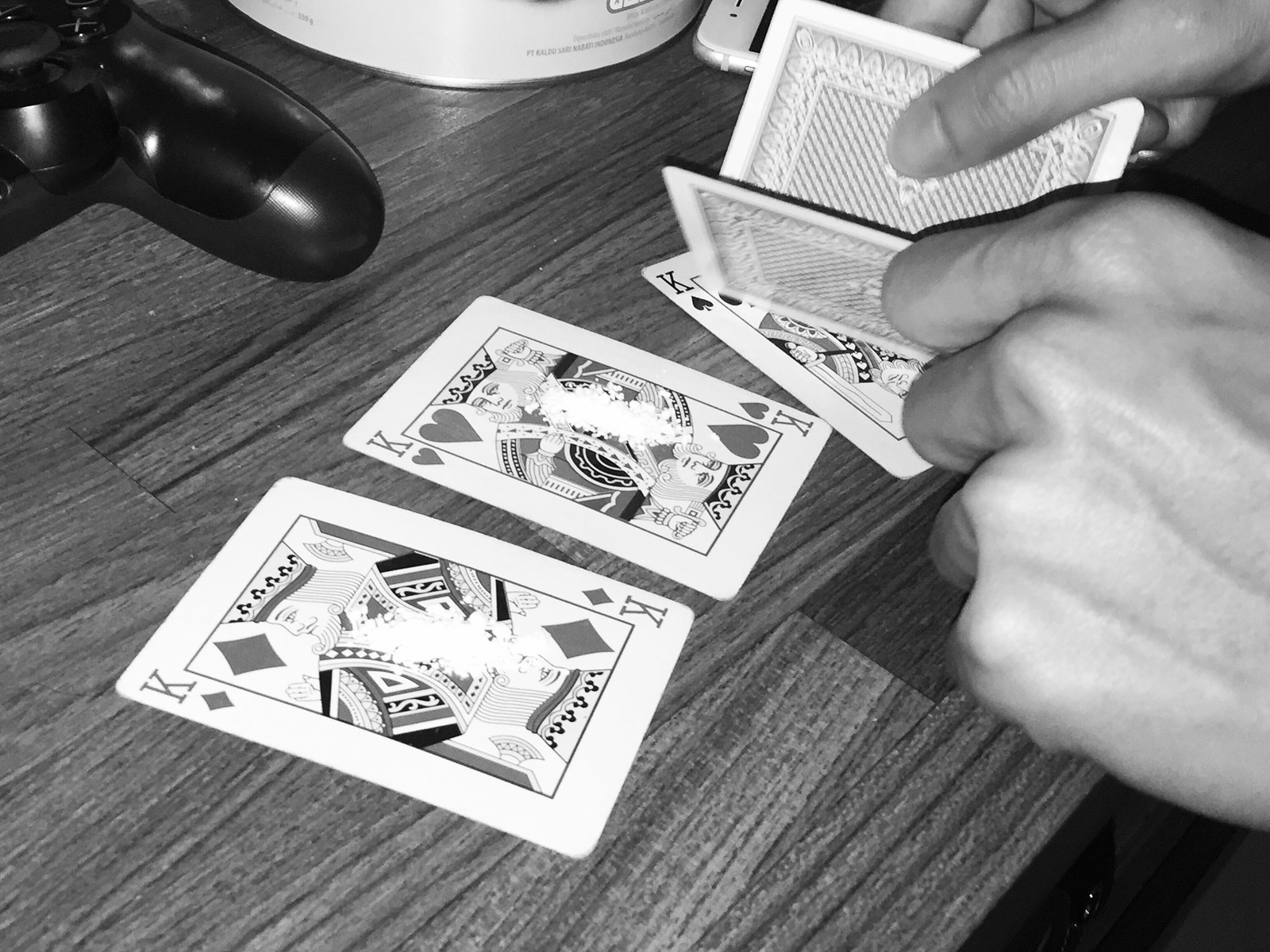A black and white photograph captures an engrossed card player, with both hands prominently positioned in the frame. The right hand is visible on the right side of the image, while the other hand appears in the upper right corner, firmly gripping a traditional deck of cards. Spread out on the table before them are three face-up King cards: the red King of Diamonds, the red King of Hearts, and a black King, their suits adding a burst of contrasts to the monochromatic scene. In the upper portion of the image, partially obscured, is the corner of an iPhone 6. Adding to the composition, the top left corner reveals half of a black gaming controller, likely for a PlayStation or Xbox. This assortment of elements weaves a narrative of focused leisure and modern-day multitasking.